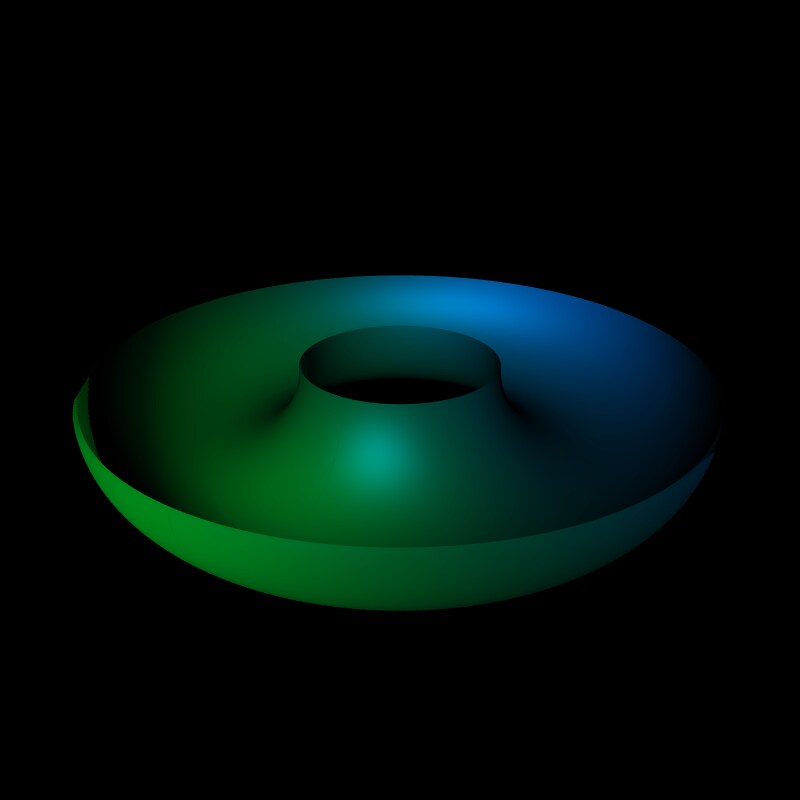The image showcases a simple 3D graphic of a pottery model, prominently highlighted in neon green and blue tones. The object has a rounded, circular structure with a hole in the center, resembling a bundt pan or a snack dish, possibly intended for holding chips or appetizers. This highlighted model sits against a stark black background, which accentuates its glowing, backlit effect, giving it a vivid and almost rainbow-like appearance. The left side of the object predominantly features green hues, while the right side is bathed in blue, creating a striking visual contrast.